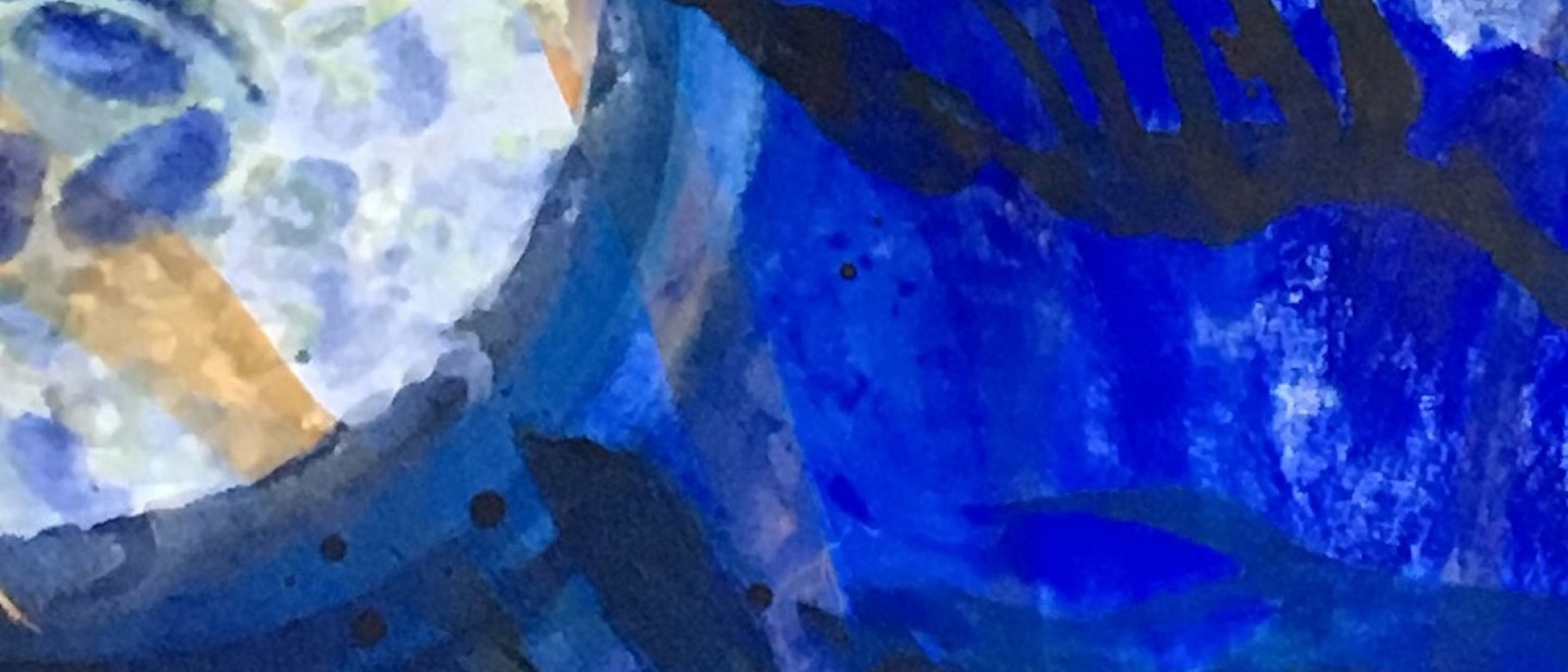This abstract painting, displayed on a long rectangular canvas, predominantly features a bluish hue with varying shades ranging from pale blue to navy blue, almost black. The piece is strikingly detailed, incorporating a background that transitions from the lighter blues to deeper blues, with sporadic touches of black and even some orange accents. On the top right, a sky blue and white blend together, while the left side showcases lighter tones with a noticeable semi-circle, resembling a sun, accompanied by blue ovals. Darker navy or black lines and dots intermittently break the continuity of the blues, adding depth and contrast. Despite the detailed elements, such as swooshes and splotches of color, the painting remains an enigmatic depiction, leaving the interpretation open to viewers. There's no text or signature from the artist, further emphasizing the abstract, exploratory nature of the work.